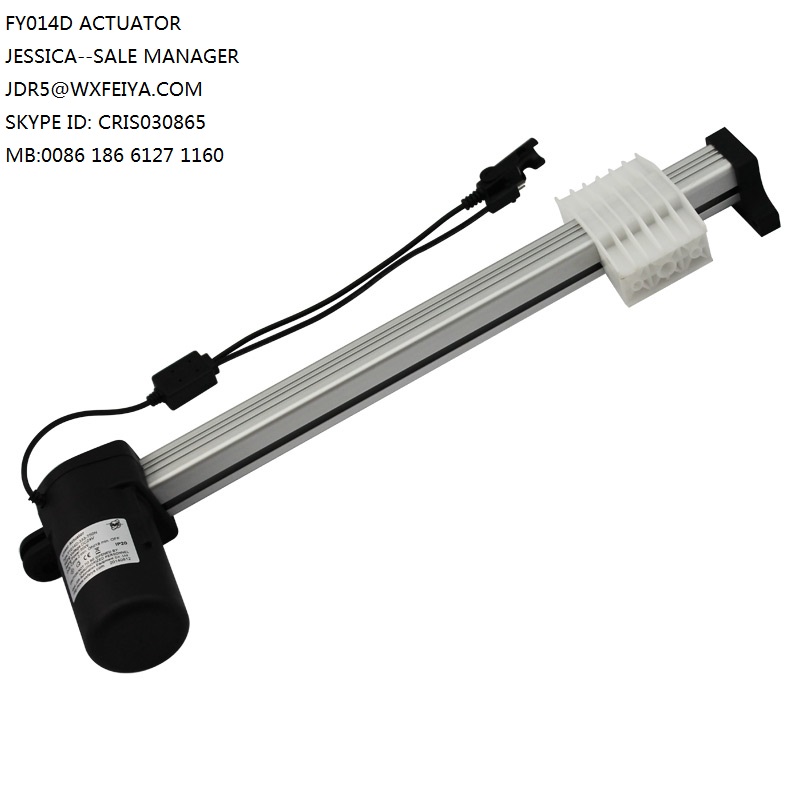This photograph prominently features a mechanical component identified as an actuator, marked by the text "FY014D Actuator" in the upper left-hand corner. Directly below this identifier, there's informative text listing "Jessica, Sale Manager" followed by her contact information, including an email address (JDR5@WX-FE-IYA.com), a Skype ID (CRIS-0308-65), and several numerical sequences, possibly related to product numbers or contact extensions (MB-0086186 61-27 11-60).

The actuator itself is a long metal bar occupying the central portion of the photograph. On one end, there is a black tube from which wires extend, splitting into two. The opposite end features a black covering, likened to the base of a lamp where a bulb would be screwed in. Affixed to the metal bar, between the two ends, is a plastic slider, which is a white clip. This detailed assembly showcases the intricate design and functionality characteristic of an actuator.